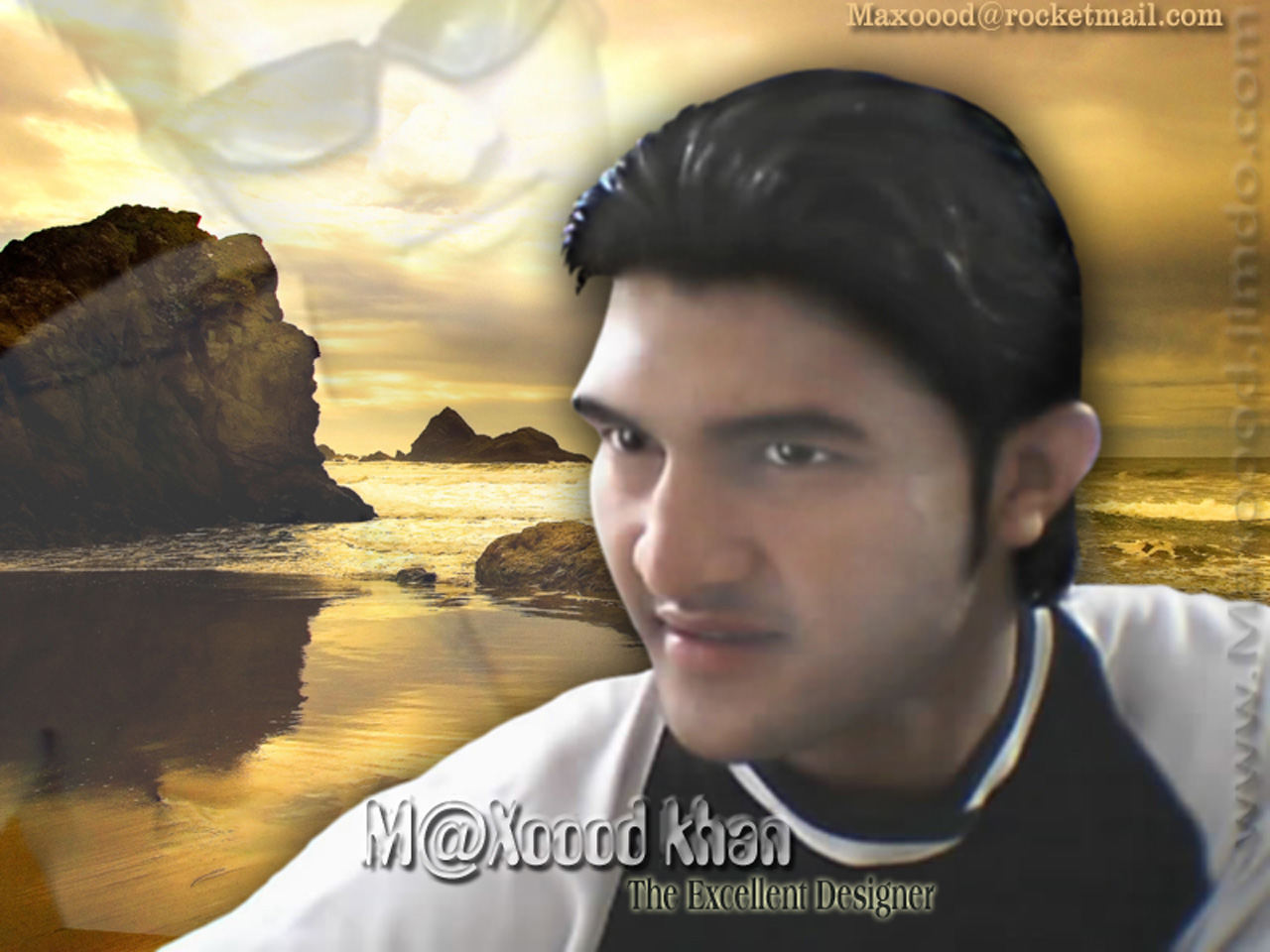The image features a vividly edited photograph of a young man with dark, gelled-up hair and long sideburns, positioned prominently on the bottom right side. He is gazing near but not directly at the camera. He is dressed in a shirt with white sleeves and a black torso. Superimposed in a translucent, ghostly fashion above him to the left is a secondary image of the same man, this time donning black sunglasses and having his head tilted.

The background sets an outdoor seaside scene with a mild tide ebbing away, revealing wet sand and a notable rock on the left. The color palette of the image includes shades of brown, tan, white, black, and gray, with an overall yellowish tint.

Text elements are abundantly present: at the top right corner, we see "maxwood at rocketmail.com" written clearly, while ascending the right side, there is partially legible text that begins with "www.maxwood.somethingdoe.com." Centered at the bottom, the image bears the caption "M@xwoodCon, the excellent designer," cleverly incorporating the "@" symbol in place of the 'a' in "maxwood." The composition suggests a creative, somewhat surreal digital design aesthetic, blending photography with graphic art, set in a natural, daytime setting.